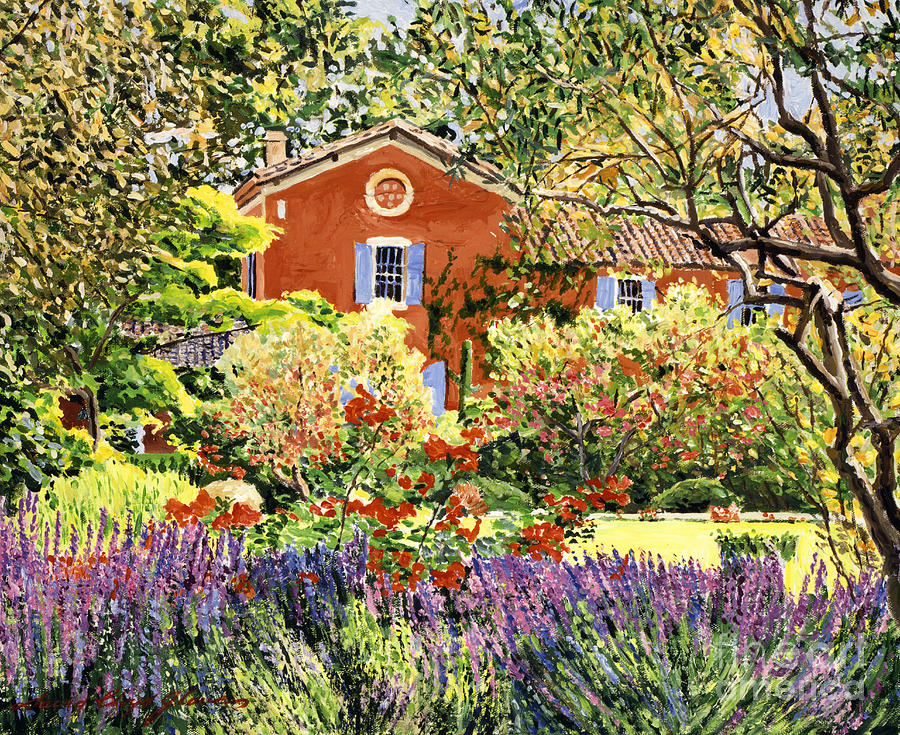This vivid painting, likely rendered in thick acrylic paint, captures a bright outdoor scene dominated by a large, red two-story house with red clay roofing tiles and purplish-blue shutters. In the foreground, lush greenery is punctuated by tall, slender clusters of purple and pink flowers, resembling lilacs, among which are dense red flower bushes. The yard is brimming with vibrant color, with patches of short, lime-green grass peeking through. The aesthetic is further enriched by trees adorned with red and yellow foliage, their texture created through splotches of thick, green paint intermingled with lighter and darker shades to provide depth and highlight. The house, reminiscent of a traditional country home, is partially obscured by this flourishing garden, drawing the eye to the interplay of colors and the suggestion of a warm, sunlit day.